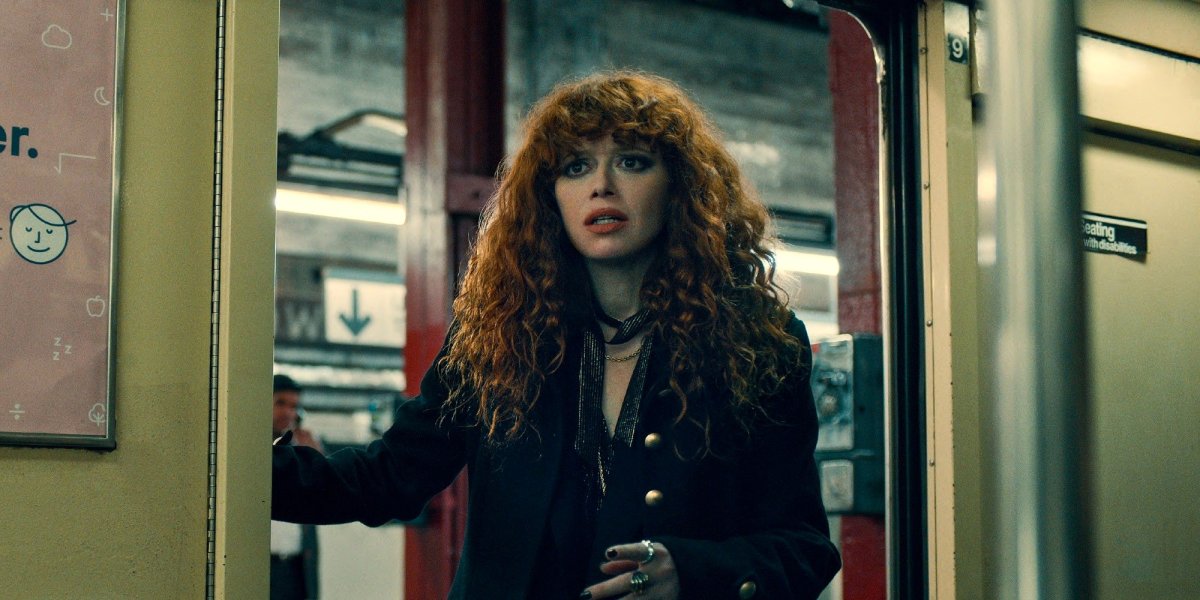The image is a detailed scene featuring actress Natasha Lyonne, likely from one of her shows such as "Russian Doll" or "Poker Face." She stands in the open doorway of a subway car, clearly identifiable with her long, wavy to curly red hair and pronounced dark eye makeup and lipstick, set against her fair skin. Natasha is dressed in a dark ensemble, including a black coat with gold buttons and a tweed blazer, and she adorns multiple rings on her fingers. Her expression seems distressed as she looks to the left. 

Behind her, the scene includes the distinctive elements of a New York City subway: red pillars, a subway pole, and other passengers. One man, blurred in the background, wears a dark overcoat and white shirt and appears to be talking on the phone. The overall tone of the image is dark with a sepia-like filter, enhancing the moody atmosphere. Additionally, the left side of the image features a barely visible light pink poster and some subway signs.